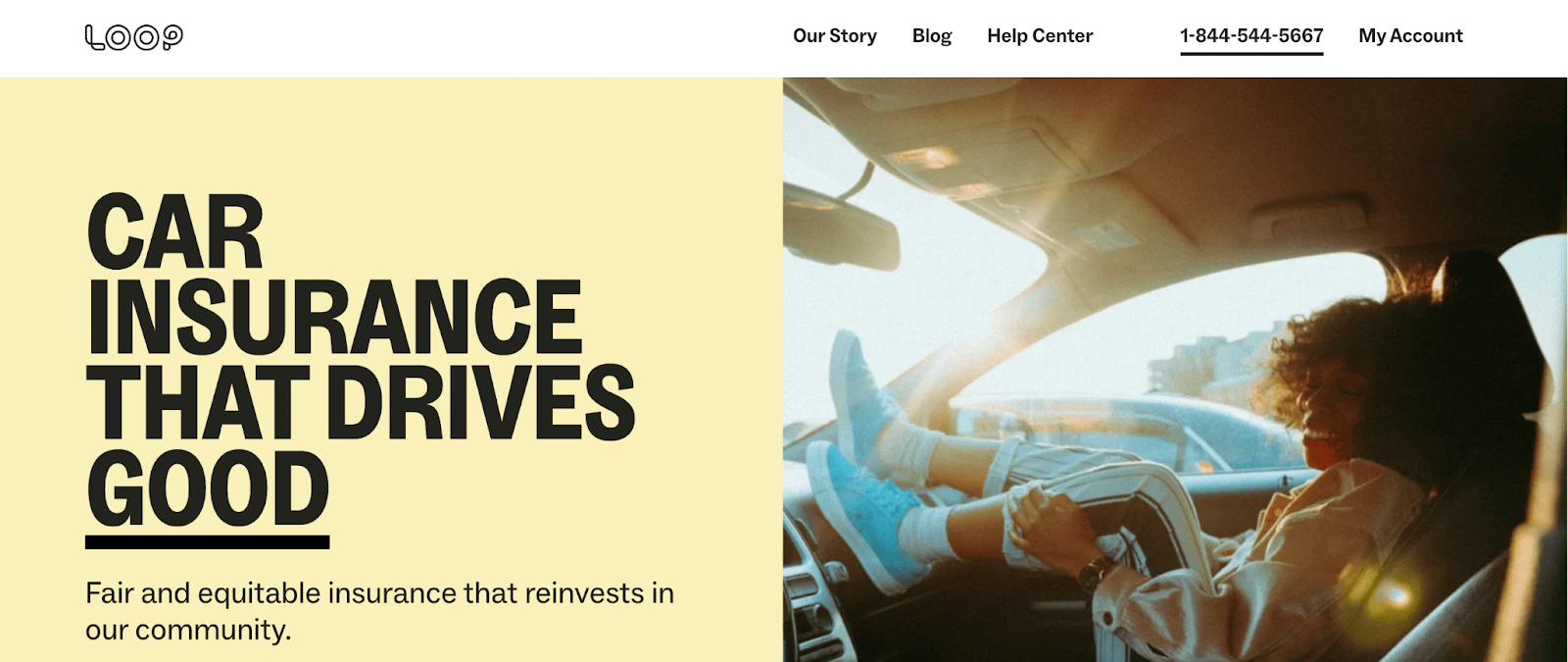In the upper left-hand corner of the image, the Loop company's insignia is prominently displayed in outlined white letters. At the top, in white, you read, "Our Story," "Blog," "Help Center," a contact phone number, and "My Account." Centrally positioned within the image is a boldly stated box with the text "Car insurance that drives good." Below this, in smaller print, it declares, "Fair and equitable insurance that reinvents our community."

On the right-hand side of the image is a woman seated in the passenger seat of a car. She's smiling and appears relaxed, with her legs slightly lifted and wearing blue sneakers. The background suggests that the car is either parked or stopped at a traffic light, evidenced by another vehicle visible beside them. The woman is dressed in a peach-colored jacket, and the photograph captures some interior details of the car, including the roof, rearview mirror, dials, and vents.

The woman is leaning back comfortably, bathed in sunlight streaming through the window, which also casts reflections on the left side, possibly bouncing off metallic elements outside. The car’s interior lights, specifically the two reading lamps overhead, are illuminated, adding a warm glow to the setting.